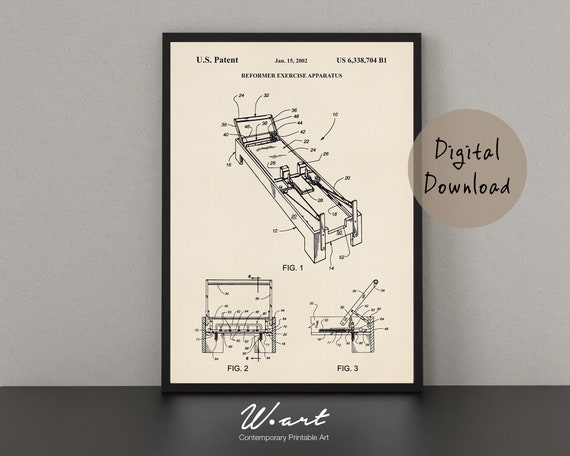The image is an advertisement for a digital download of contemporary printable art, specifically showcasing a U.S. patent for a Pilates reformer exercise apparatus. The central focus is on a detailed drawing from the patent, dated January 15, 2022, featuring the apparatus' various components. The patent number is situated in the upper right corner, while the words "US patent" are prominently displayed in the upper left. The diagram is divided into three views: an overall top view (Figure 1), an angled view (Figure 2), and a side view (Figure 3), with Figures 2 and 3 smaller and positioned at the bottom of the patent sheet. The apparatus itself is long and rectangular, detailed with labeled numbers and letters outlining its different parts and mechanics.

The advertisement page includes a tan bubble on the right side, indicating the availability of a digital download in stylized cursive text. The background of the patent drawing is white, bordered by a black trim, enhancing its appearance as a piece of wall art. The entire image rests against a vertical gray surface, possibly mimicking the look of it being hung on a wall, and it sits atop a dark-colored, marble-like floor. Below the patent diagram, the text reads "W Art, Contemporary Printable Art," marking the seller and the nature of the product. The overall color theme is a mix of light tan and grayscale, giving it a vintage and professional look.